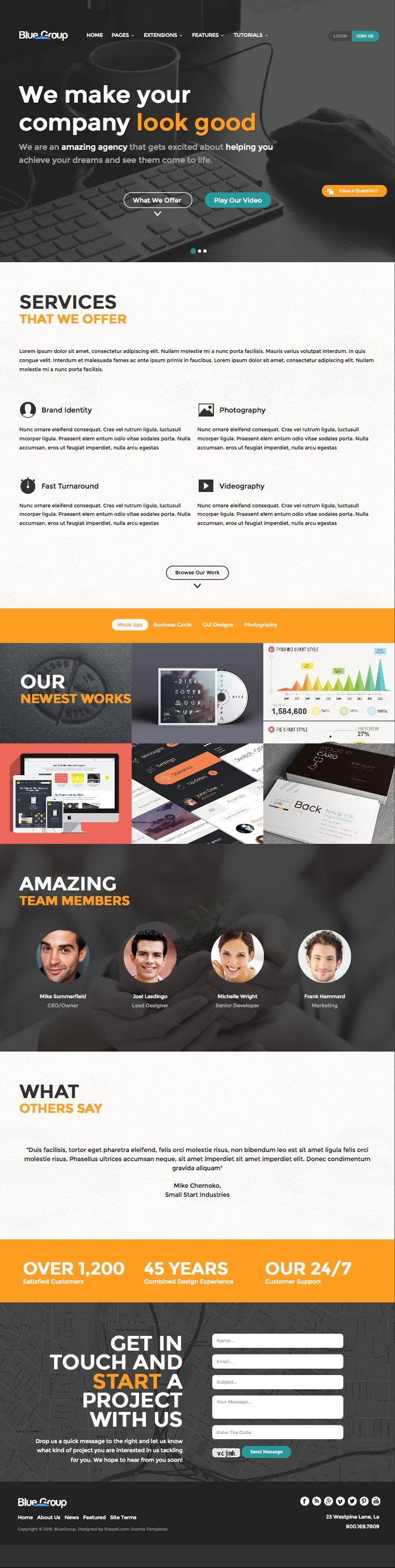**Caption:**

The image captures a detailed screenshot of a B2B marketing agency's homepage, designed to showcase their comprehensive services and expertise. Starting with a striking banner image that boldly declares, "We Make Your Company Look Good," the homepage immediately invites users to explore further through strategically placed buttons leading to more information about their offerings.

Following this introduction, the next section highlights the agency's core services under a banner titled "Services We Offer." Here, potential clients can learn about the various services provided, including brand identity, photography, videography, and more, all promising a fast turnaround.

The homepage then transitions into a showcase of sample marketing materials created by the agency, including a CD jacket, data visualizations, business cards, and various webpage designs, giving visitors a concrete sense of their creative capabilities.

In the "Amazing Team Members" section, the agency introduces four key team members with professional photographs, names, and job titles, adding a personal touch and illustrating their expertise.

Further down, the "What Others Say" segment features a testimonial endorsement and impressive statistics: over 1,200 satisfied customers, 45 years of experience, and 24-7 availability, underscoring their reliability and customer satisfaction.

Finally, the homepage concludes with a "Get in Touch and Start a Project with Us" contact form, encouraging prospective clients to reach out, accompanied by a basic website footer for additional navigation.